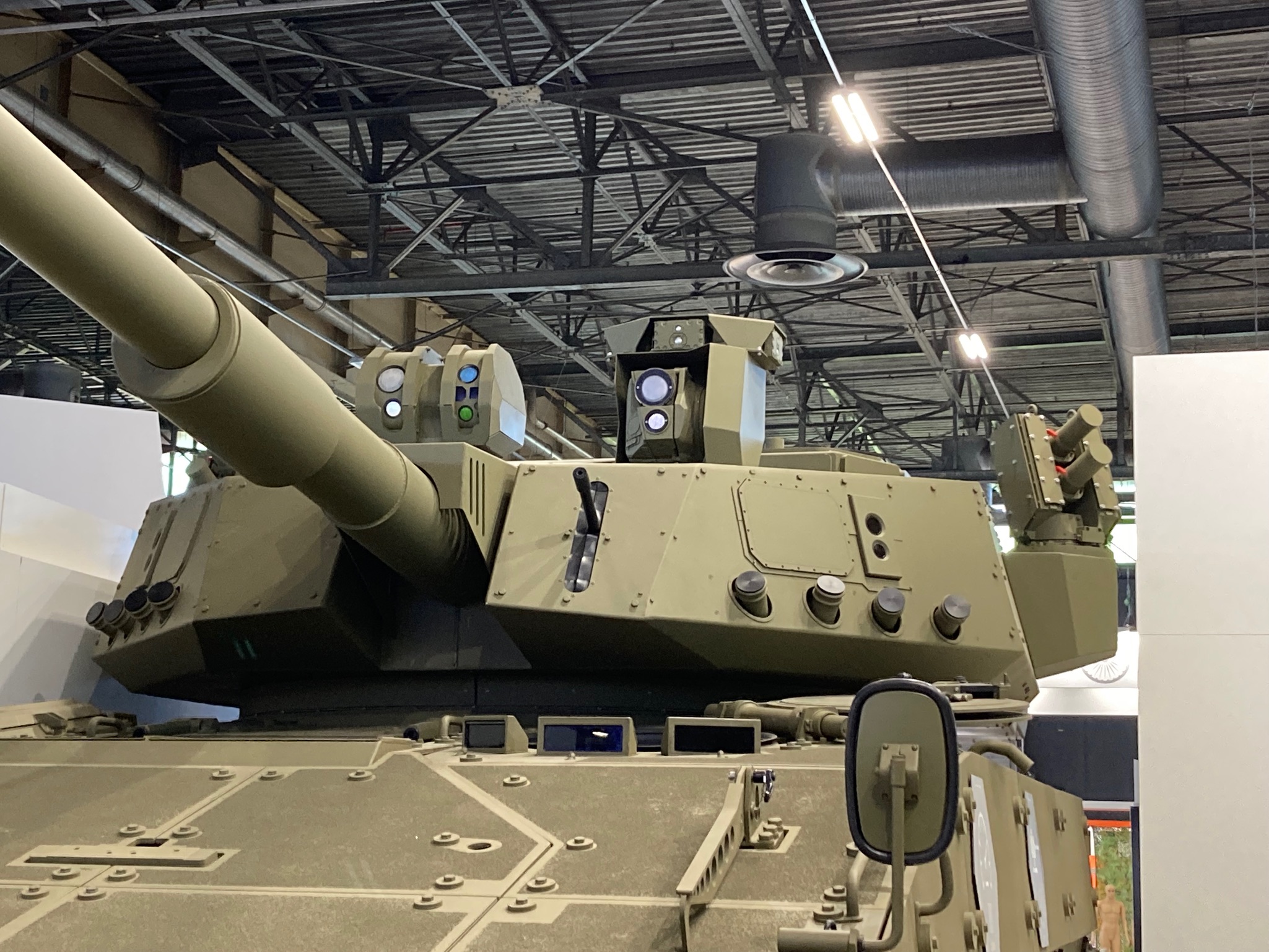The image is a square, close-up shot of a military tank situated within a warehouse-like facility. Dominating the frame is the front side of the tank, which features a brown hood with light brown trim. Several circular lenses adorn the tank’s surface—some being clear, with one blue and another green. In addition to numerous knobs and what appears to be a shifting stick, a mirror is positioned towards the bottom right of the tank. The tank’s cannon protrudes and angles towards the upper left of the image. The surrounding environment is characterized by a ceiling filled with an intricate network of metal bars in various directions, along with fluorescent lights attached to white poles, contributing to the industrial feel of the scene.